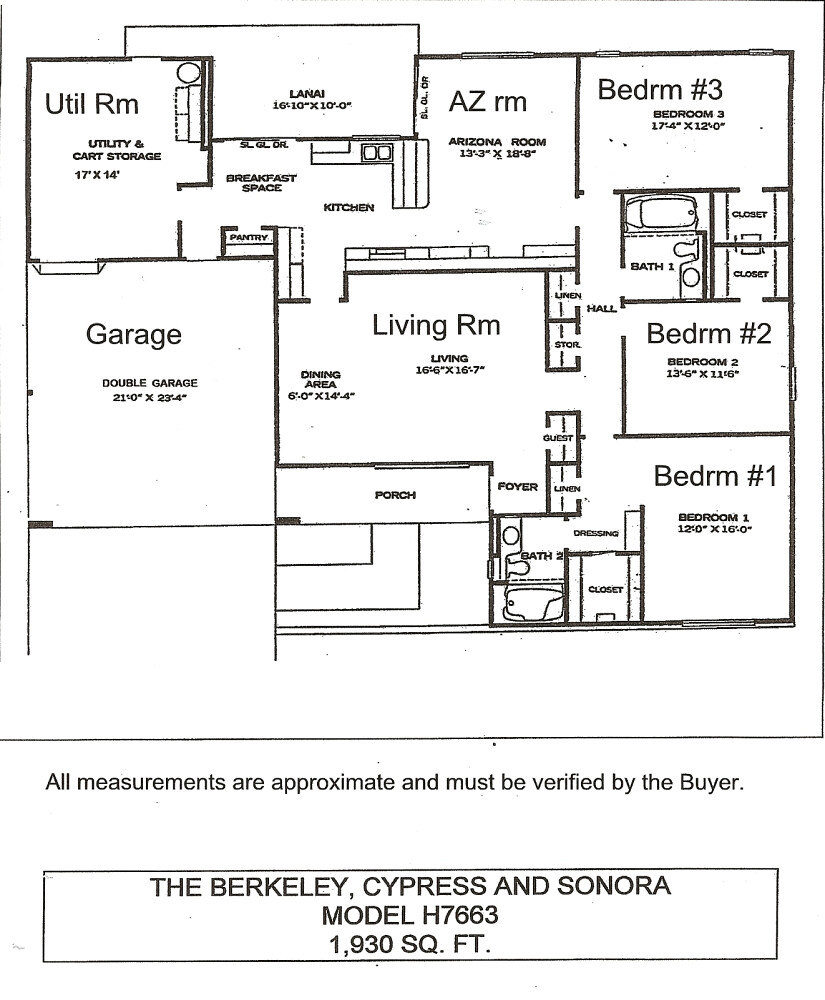The image showcases a scanned blueprint of a single-story, ranch-style residential home, distinctly laid out on a white piece of paper. This detailed floor plan, titled "Berkeley, Cypress, and Sonora, Model H7663," represents a 1930-square-foot house. A note on the blueprint states, "All measurements are approximate and must be verified by the buyer."

The layout is quite square, with a balanced and practical design. On the left side, the blueprint features a utility room adjacent to a designated space for a garage. The right side of the home is organized with three bedrooms aligned in a single column, labeled "Bedroom 1," "Bedroom 2," and "Bedroom 3." The central area houses the living room, which opens to a porch via an indicated door. Additionally, the floor plan includes two bathrooms and a modest kitchen, suitable for an efficient and cozy living space. The utility and garage space enhances the home's functionality, making the blueprint a comprehensive guide for prospective buyers.